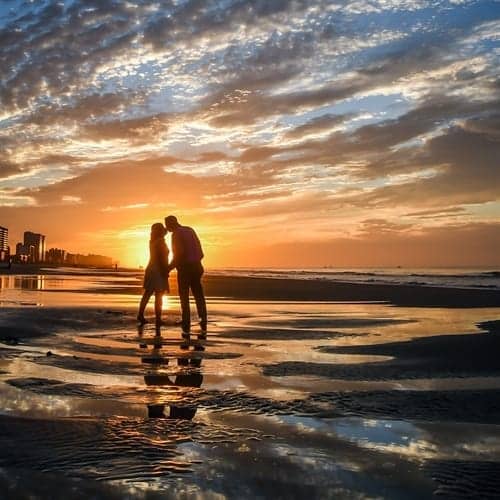In this mesmerizing beach scene, a couple shares a romantic kiss amidst a stunning sunset. Positioned centrally, with the woman on the left and the man on the right, they stand at the water's edge where small, gentle waves have formed reflective puddles in the sand around them. The sunset casts a radiant orange and red glow across the partially cloudy sky, with hints of blue and gray peeking through. The reflection of the vibrant sky and the sun can be seen shimmering in the puddles at their feet. In the background, to the left, the silhouettes of tall buildings and possible trees form a cityscape, while a couple of distant boats are visible on the ocean. The overall atmosphere exudes romance and tranquility, enhanced by the soft evening light enveloping the couple in a semi-silhouette as they embrace on this magical evening.